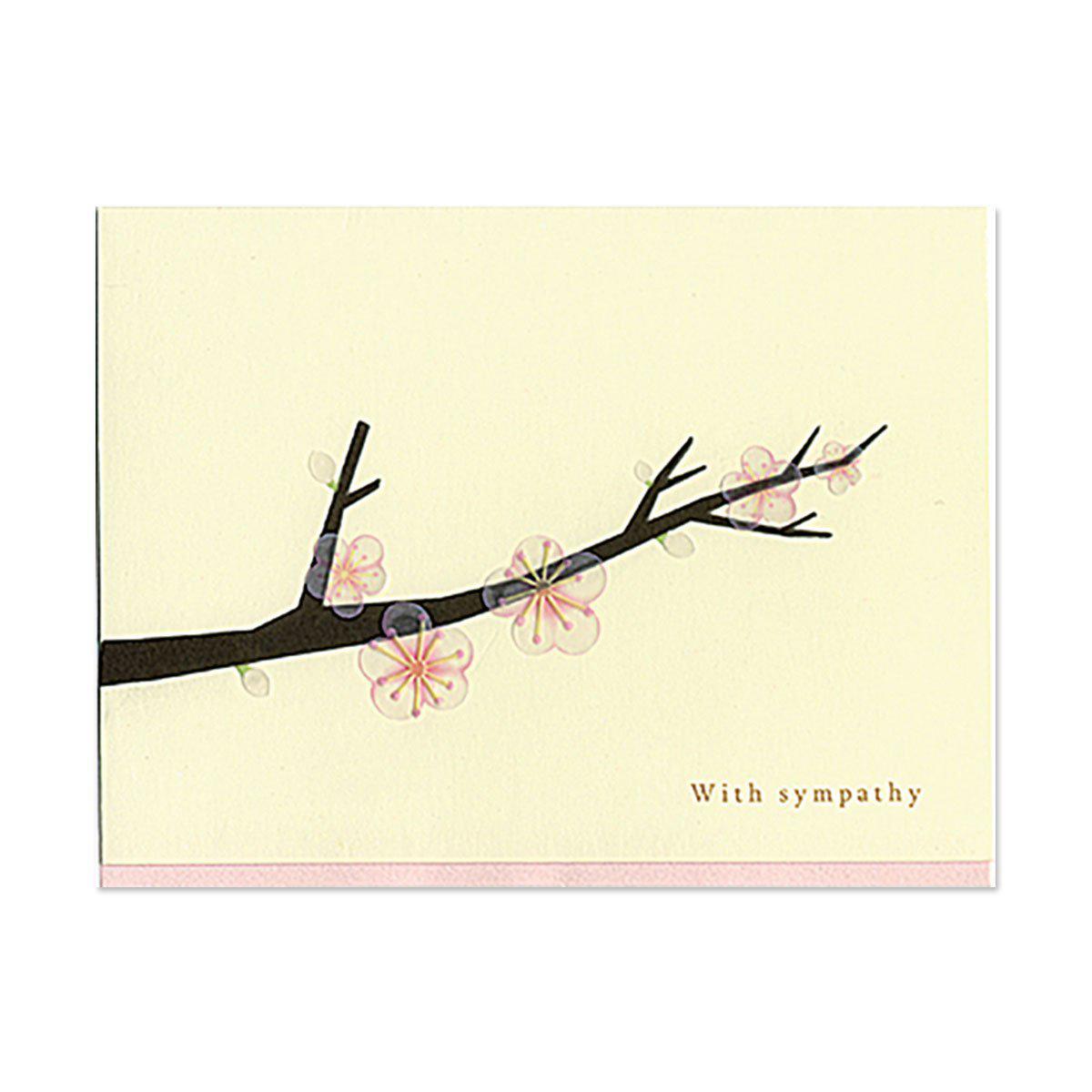The cover of this sympathy card features a soothing, creamy yellow background, enhanced by a light pink strip running horizontally along the bottom. In the lower right-hand corner, the words "With Sympathy" are elegantly inscribed. A dark brown, almost blackish tree branch extends nearly all the way across the card from the left side, giving a sense of gentle movement. The branch is adorned with several ornate and puffy translucent flowers in shades of pink, fewer than a dozen, each intricately detailed with gold accents radiating from their centers in a starburst pattern. Sprinkled among the flowers are a few tender buds and a handful of faint green leaves, adding subtle, delicate touches to the scene.